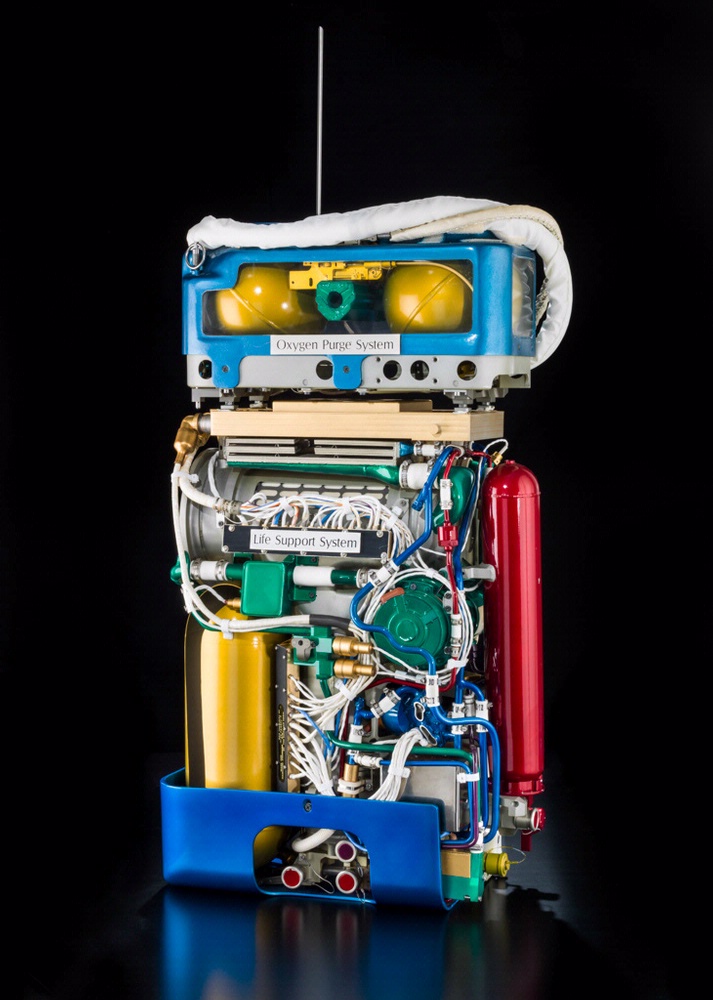A meticulously crafted robot sculpture stands against a stark black background, showcasing an assemblage of circuit boards and computer innards. The robot’s head, encased in a blue rectangular shell with silver accents, features round gold balls for eyes, giving it an uncanny semblance to a face. Wrapped white cables cascade around its head, resembling hair. Its exposed body reveals an intricate network of wires, circuit boards, and various other computer components, lending the figure a raw, mechanical aesthetic. A red arm extends from its side, adding a striking contrast to the otherwise metallic palette. The overall creation, though not lifelike, evokes a fusion of technology and imaginative artistry.